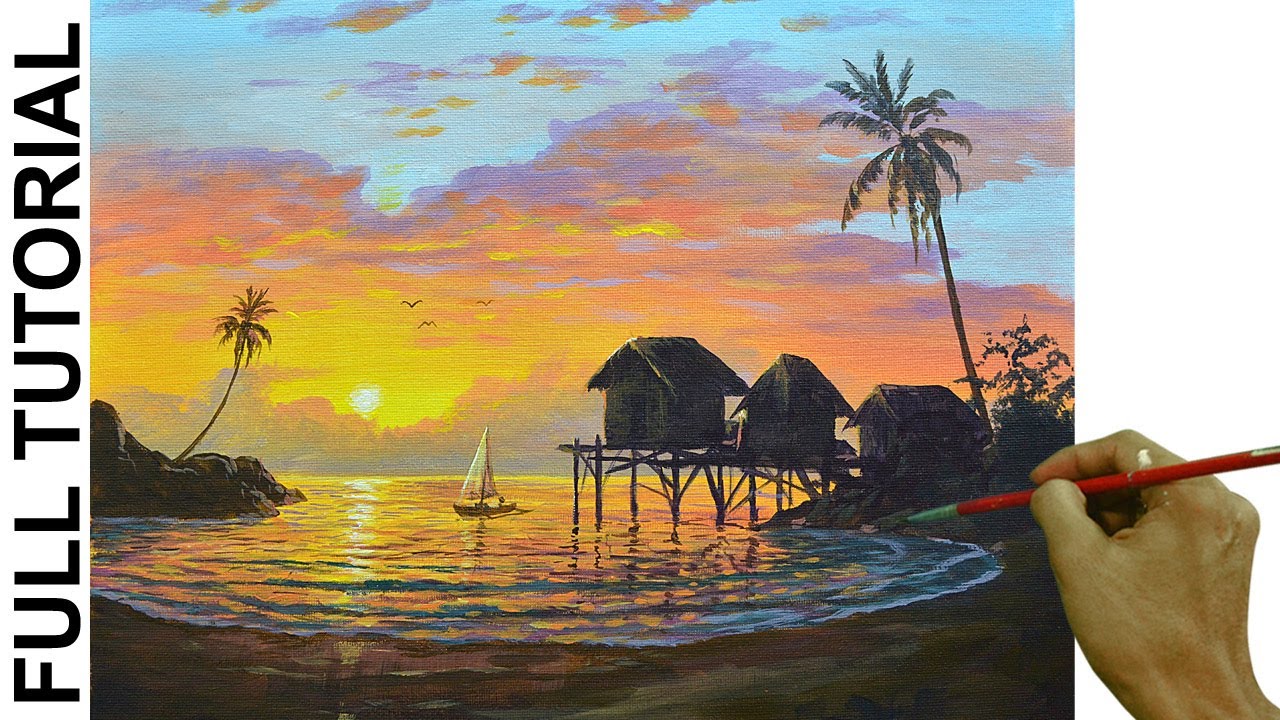This image showcases a detailed and colorful tropical sunset scene, likely included in a home "teach yourself how to oil paint" kit. On the left side of the image, the vertical text on a white background reads "full tutorial." Dominating the center, the painting features a striking sunset with a fiery blend of reds, oranges, and yellows accenting the sky, along with purples and blues. A small island with a lone pine tree juts into the water on the left, while on the horizon, three rustic grass-roofed huts stand on stilts, flanked by a leaning, towering palm tree on the right. Nestled between the island and the huts is a small sailboat, floating in the sunlit inlet. In the bottom right corner, a light brown hand delicately holds a red-handled paintbrush, touching up the vibrant scene, adding a personal touch to the idyllic, serene seascape. The meticulously depicted reflection of the setting sun shimmers across the water, enhancing the tranquil beauty of this artistic composition.